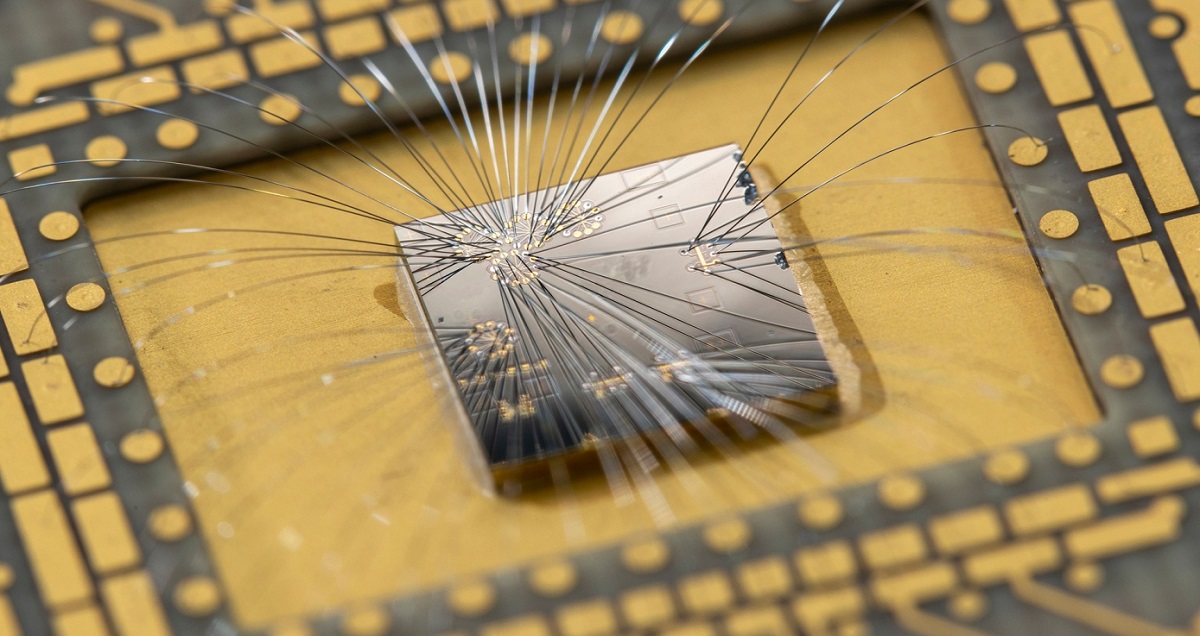The image is a close-up photograph of a computer chip or processor. At the center is a shiny, metallic square, silver with a black tint, which is likely the main processing unit. From various parts of this central square, numerous super tiny, black, thin wires extend outward. These wires are connected to golden dots and circles on the central unit, forming intricate patterns. Surrounding this central metallic area is a recessed, yellow rectangular zone. Outside of this yellow rectangle lies a dark gray PCB board populated with golden circles and square-shaped contact pads. These pads and circles are uniformly distributed around the central unit, and the wires from the central silver square connect to these pads on all sides—top, bottom, left, and right—creating an intricate network. The overall layout is highly detailed, showcasing the complex design of the circuitry.